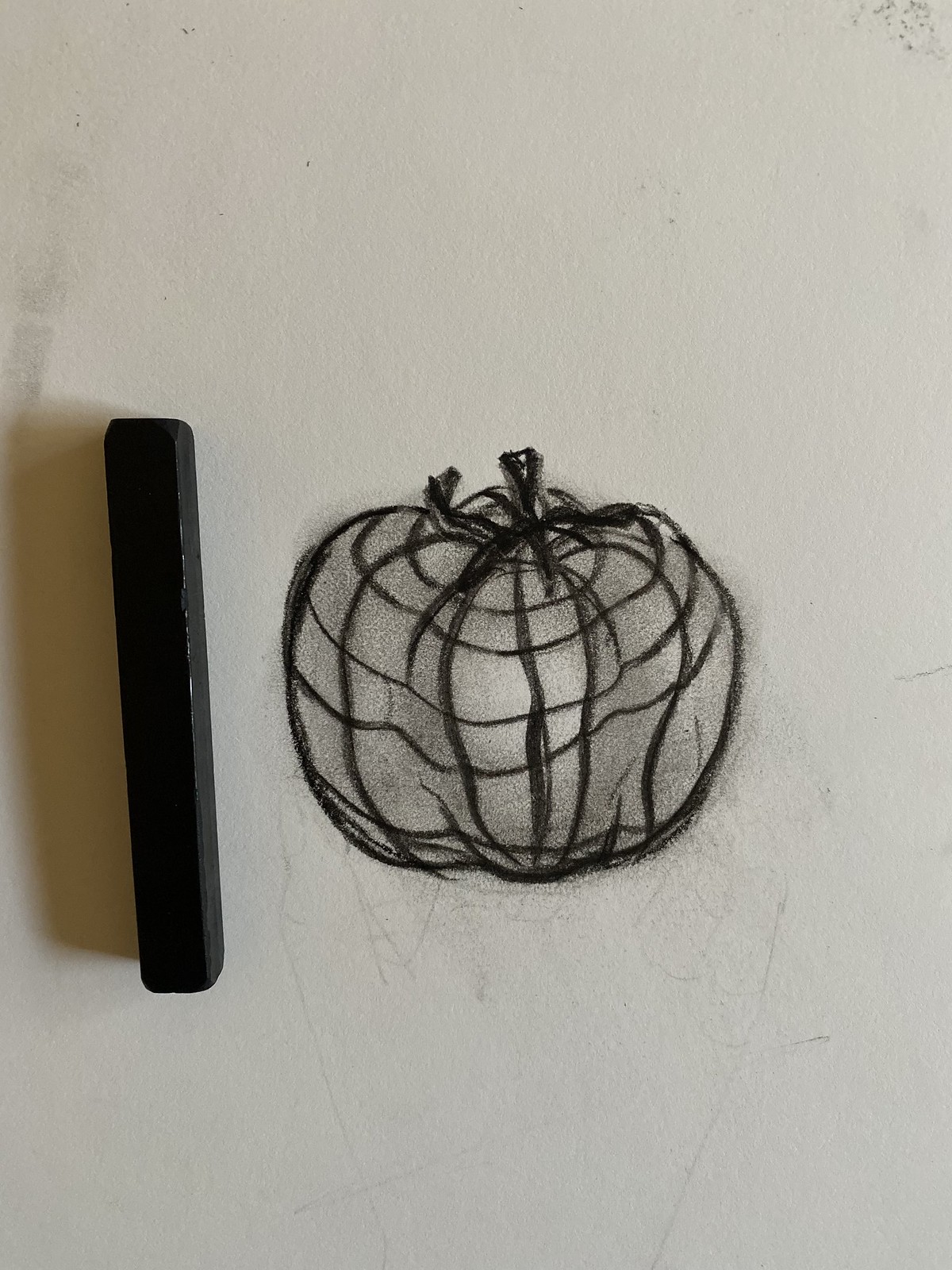This photograph captures a detailed charcoal drawing on a white sheet of paper, viewed from above in a portrait orientation. At the drawing's center, slightly to the left, there's a rectangular stick rendered in deep black, demonstrating a three-dimensional quality suggestive of a square or rectangular column. This stick casts a pronounced shadow to the left, extending to the edge of the paper.

Central to the composition is a meticulously sketched pumpkin, characterized by its rounded form and outlined in dark black. The pumpkin's short, dark stem crowns the top, while curved lines depict its lobed surface, giving the gourd a realistic texture. Additional detailing includes lateral curved lines that enhance the pumpkin's dimensionality. The shading is expertly handled, with lighter tones in the middle that gradually darken toward the edges, emphasizing the pumpkin's form and volume. The use of monochrome shades of black and gray lends the drawing an elegant and timeless quality.